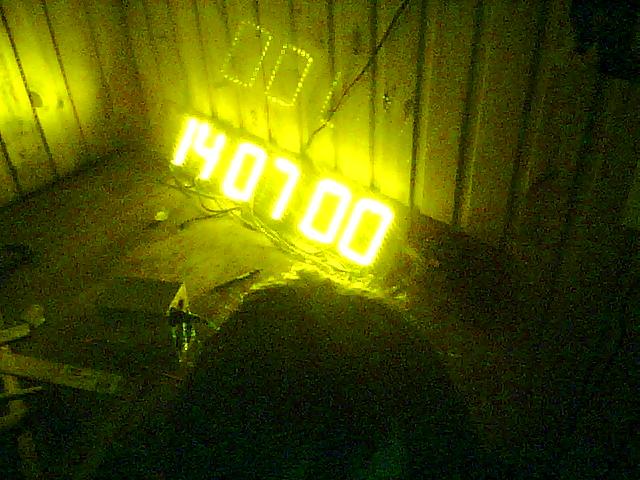In this grainy, low-light photograph, the foreground is dominated by illuminated neon green LED digits that display the number "140700." These glowing numbers are mounted on a wall made up of wooden planks and beams, adding a rustic texture to the scene. Below the wall sits a metal or electric box, which appears to be some sort of charging generator with wires trailing up to the illuminated digits, suggesting a possible power source connection. The entire image has an old, cloudy, and grey appearance, indicative of it being taken with an outdated camera, possibly from the early 2000s. The photograph is further marred by strange indentations and marks on the walls, contributing to the enigmatic and aged atmosphere of the scene.